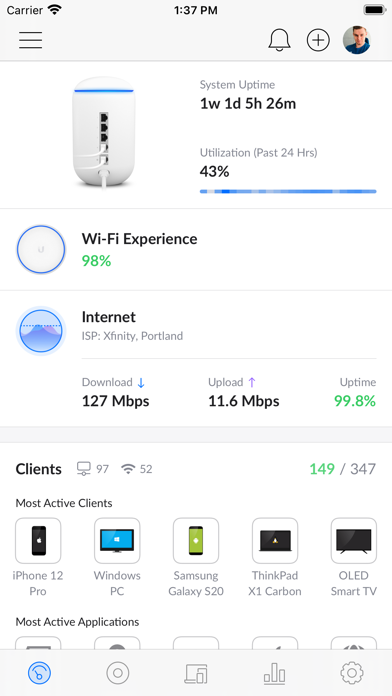The image shows a detailed screenshot from a smartphone, displaying what appears to be a network monitoring interface. At the top, there is a device depicted, likely a router or network hub, which supports multiple connections. The interface indicates the system has been running for a duration of one week, one day, five hours, and 26 minutes. 

Utilization over the past 24 hours is captured, showing an average of 43%, represented visually by a horizontal bar graph featuring alternating strips of gray, blue, and dark blue. 

Further down, under "Wi-Fi Experience," there is a circular icon with a white background, a blue outline, and a letter "U" in the center. The performance metric here shows 98% in green text. 

The section labeled "Internet" follows, displaying another circular icon and details about the internet service provider, Xfinity Portland. It reports a download speed of 127 Mbps, an upload speed of 11.6 Mbps, and an impressive uptime of 99.8%, all highlighted in green.

At the bottom, there is a "Clients" section, indicating that 149 out of a possible 347 clients are currently connected, with the number 149 shown in green.